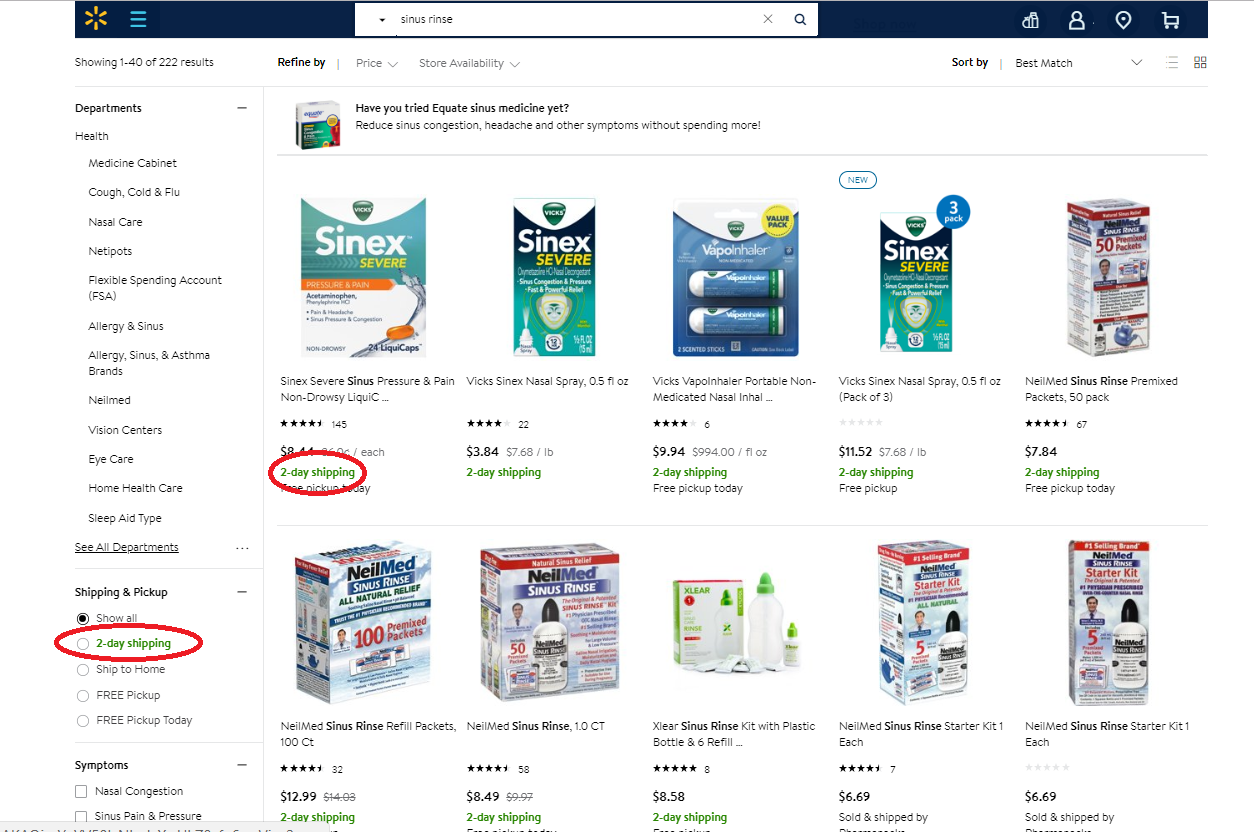This image features an online storefront belonging to Walmart, distinguishable by the yellow insignia resembling a flower with radiating petals in the upper left corner. On the left side, three horizontal blue lines are visible, indicating a menu or navigation option. The interface includes a prominent black header bar across the top, within which a search bar contains the query "sinus rinse." To the right of the search bar are various icons, including an empty shopping cart icon.

Beneath the header, the page falls under the "Health" category, displaying subcategories such as Medicine Cabinet, Cough, Cold & Flu, Nasal Care, Neti Pots, Flexible Spending Account, Allergy & Sinus, Allergy, Sinus & Asthma, Neti Med, Vision Centers, Eye Care, Home Health Care, and Sleep Aids. There is an option to "See All Departments" in black, underlined text. Additionally, the page offers sorting options with selections for "Shipping," "Pickup," and an “All” option.

A user has circled "Two-Day Shipping" in green text with a red marker. Under the shipping options, there are symptom-specific sections listed as Nasal Congestion, Sinus Pain, and Pressure. Featured products below this section include approximately ten items with their prices displayed. Among these, a Vicks Sinex Severe product with two-day shipping highlighted is specifically circled, and a blue-highlighted price of approximately "three something" is attached to the Vicks Sinex Nasal Spray.

This detailed and descriptive caption effectively illustrates the content and layout of the Walmart online store page focused on health-related products, particularly those for nasal and sinus care.